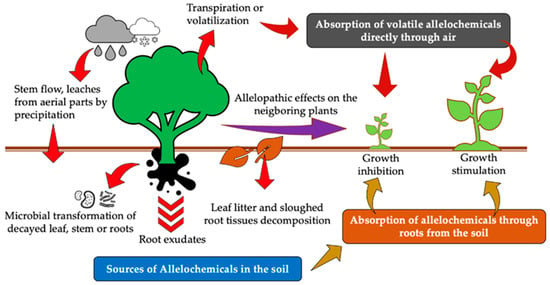This detailed diagram illustrates the science of allelochemical interactions in nature. At the center, a tree resembling broccoli stands prominently, with its roots and surrounding environment depicted in a black blob. Above the tree, a small grey cloud and a white cloud appear to rain down on it. 

A purple arrow extends to the right from the tree towards a small sprout emerging from the ground, next to which is a larger sprout, showing stages of growth. The diagram is heavily annotated with red arrows pointing to various text labels and text boxes, explaining the processes.

The key annotations are:
- "Sources of allelochemicals in the soil" below the black blob.
- "Absorption of volatile allelochemicals directly through air" in a top right text box.
- "Absorption of allelochemicals through roots from the soil" in an orange text box on the bottom right.
- "Stem flow leaches from aerial parts by precipitation," indicating the role of rainfall.
- "Microbial transformation of decay leaf stems of roots goes into the growth of the tree."
- "Transpiration or volatilization" at the very top shows the process of allelochemicals moving through the atmosphere and affecting other plants.

This cohesive visual representation highlights the complex interactions between precipitation, microbial transformations, and the absorption of allelochemicals through various pathways, ultimately demonstrating the chain of growth and simulation in nature.